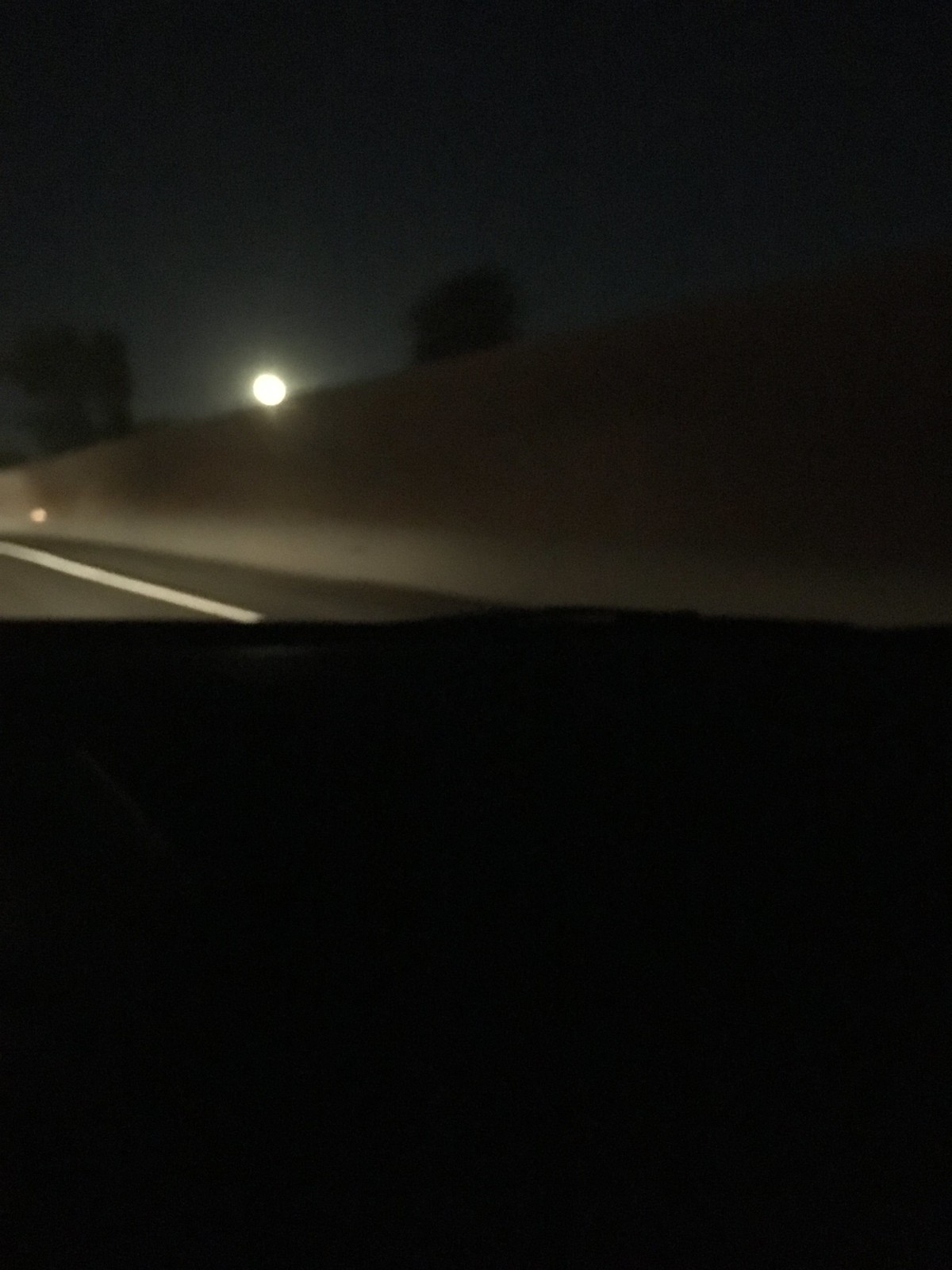A captivating nighttime image, possibly captured from inside a vehicle or behind a wall, features a mysterious black section at the bottom resembling part of a car. Just above this black area, the image showcases a stretch of gray asphalt, accented by a crisp white line delineating its edge. Beyond the asphalt lies a light brown sandy hill, gradually ascending to reveal a few scattered trees. The image fades into deep darkness at the right edge of the hill, with the most prominent light source being a luminous, white moon rising majestically over the hill's crest, casting a serene glow over the scene.